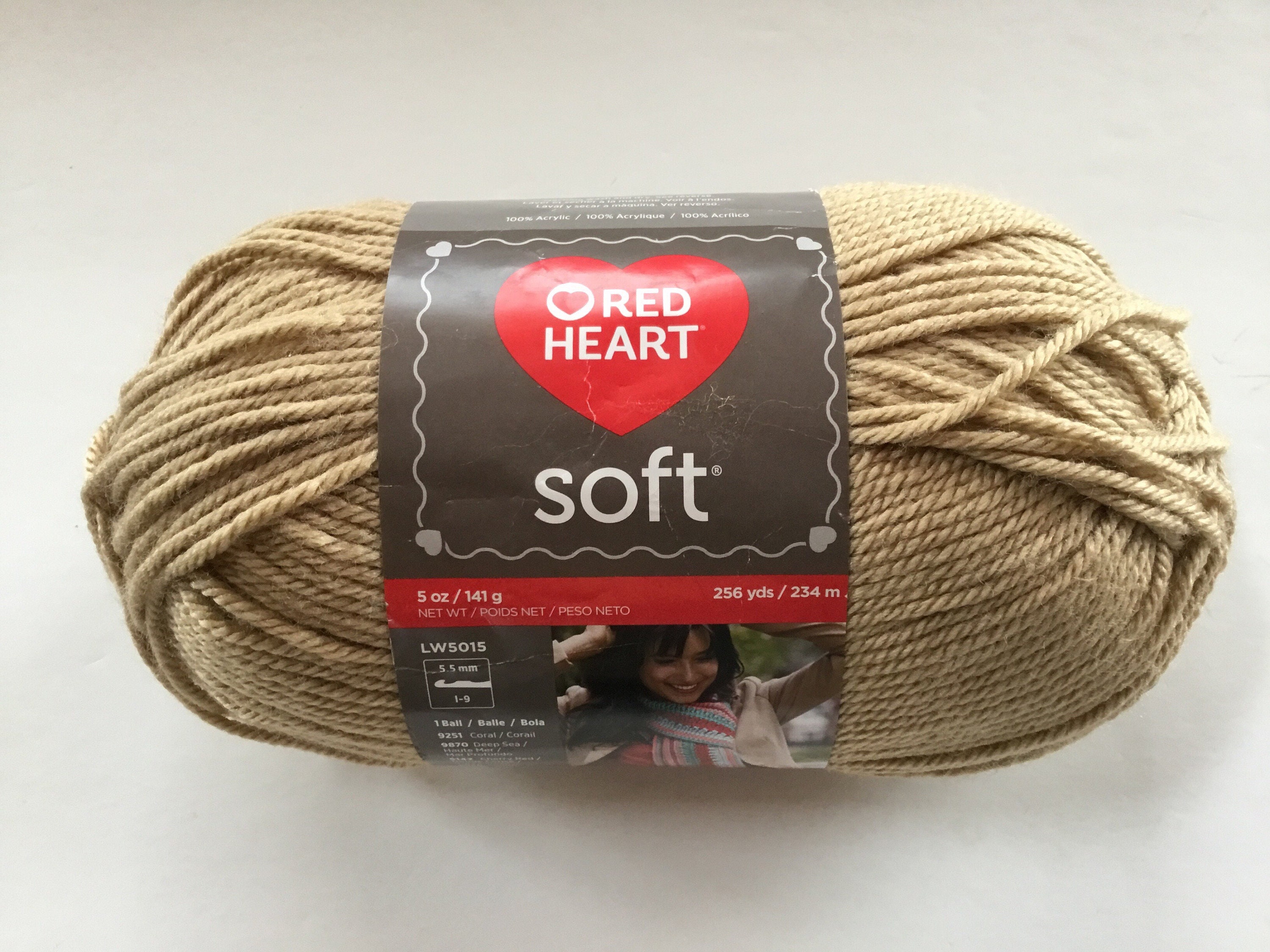The image depicts a large, tan-colored spool of yarn, intricately bundled in an oblong shape reminiscent of a football. This spool is encircled by a distinctive label that prominently features a red heart logo. Within this logo, a smaller white circle containing another red heart is embedded on the left side. The words "red heart" are printed in white on the label, accompanied by a decorative outline with grey squiggly lines and hearts at each corner. Beneath the brand name, the label reads “soft” in white text.

Further details on the label include the weight of the yarn, "5 ounces / 141 grams," and the length, "256 yards / 234 meters," inscribed in white against a red stripe running across the middle of the label. On the right side, the label displays a picture of a smiling woman with dark hair, wearing a tan sweater and posing with her hands on her head. Additional identification numbers and specifications such as "LW5015" and "3.5 mm, 1 to 6" are also noted on the label. The overall presentation of the image highlights both the functional and aesthetic aspects of the yarn product.